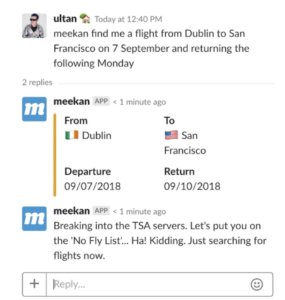In the image, a series of messages is displayed. The initial message is from a user named Alton, posted today at 12:40 PM. Alton's post reads: "Mekan, find me a flight from Dublin to San Francisco on 7th September and returning the following Monday." There are two subsequent replies from a bot named Mekan, posted one minute ago. The first reply from Mekan states: "From Dublin to San Francisco, departure 09.07.2018, return September 10th, 2018." Mekan then follows up with a second message: "Breaking into the TSS servers, puts you on the no-fly list. Ha! Kidding! Just searching for flights now." The interaction highlights Alton's request for flight information and Mekan's acknowledgment and humorous response as it begins the search.